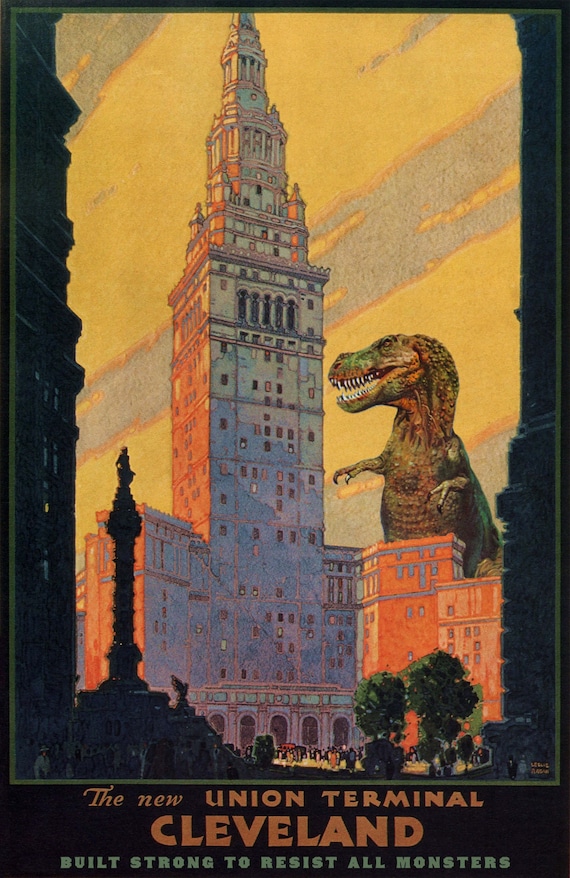This vintage movie poster is a detailed, vivid depiction of a fantastical scene centered around the New Union Terminal in Cleveland. The primary feature is a towering high-rise terminal, around 70 stories tall, standing majestically against a striking yellow sky streaked with blue and gray clouds. The building itself is a pristine white, adorned with ornate domes at the top, and framed by shadowy silhouettes of other buildings that simulate a tunnel view.

Prominently, the right side of the scene is dominated by an ominous T-Rex, its orange and gold scales glinting sinisterly, and its dark green highlights giving it a fearsome appearance. Its mouth is slightly open, revealing its sharp white teeth, as it looms menacingly near the high-rise, almost three-quarters the height of the building. Below, clustered at the base, minuscule human figures add a sense of scale to the gigantic creature and the towering structure.

To the side, orange lower-rise buildings contrast with the dominant high-rise. Details include dark green and black trees and a statue on the left, fitting seamlessly into the colorful, watercolor-like aesthetic of the poster. At the bottom of the image, bold red letters on a black background read, "The New Union Terminal, Cleveland," with green text underneath stating, "built strong to resist all monsters," emphasizing the terminal's supposed resilience against even the most formidable of creatures.